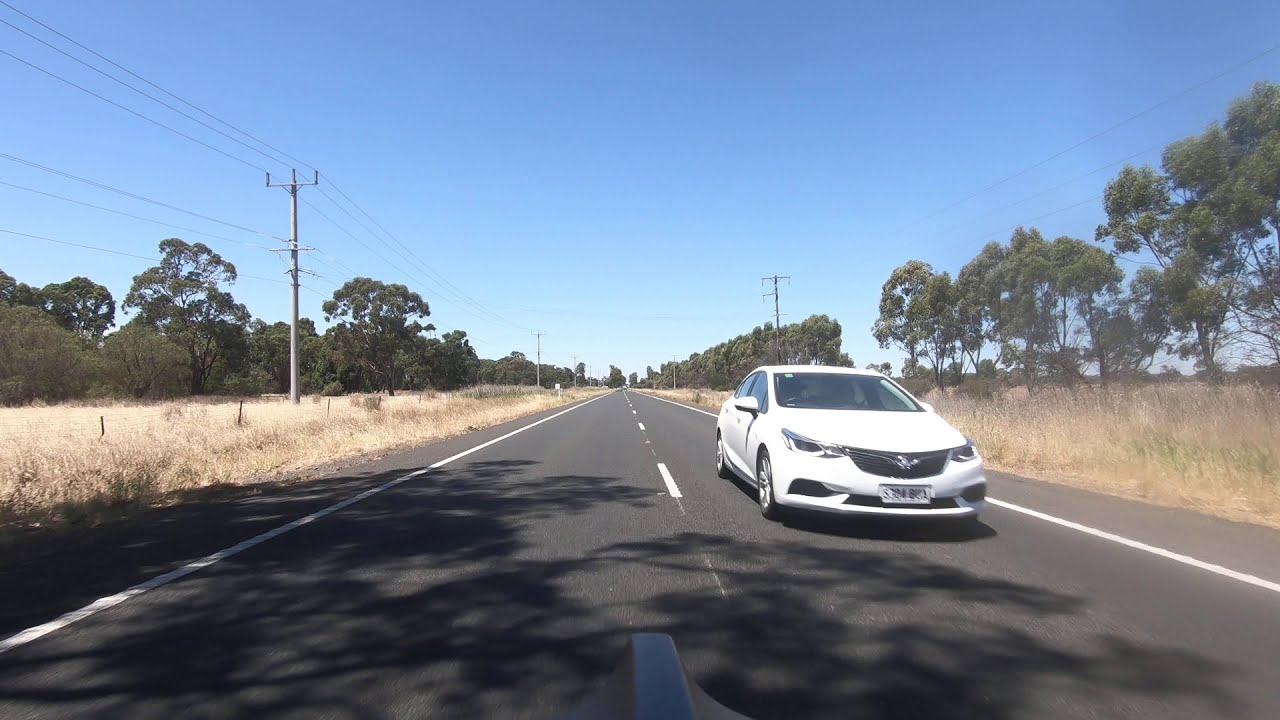This horizontally aligned rectangular photograph captures a clear blue sky over a two-lane, nicely paved gray road adorned with a dashed white line down the middle and solid white lines on each side. A white sedan, unidentified by make, is approaching in the right lane, showcasing a front license plate whose numbers are indistinguishable due to distance. The landscape on both sides of the road features tall, dried, brown grass and rows of lush green trees, with power lines and poles lining the horizon. A small, hard-to-identify plastic object, possibly a part of a vehicle or motorcycle, appears at the very bottom center of the image, suggesting the photographer is likely in their own vehicle. In the distant background, a faint, indiscernible spot hints at another vehicle. The scene is lit by the sun, casting some shade over parts of the road, emphasizing the serene, cloudless day.